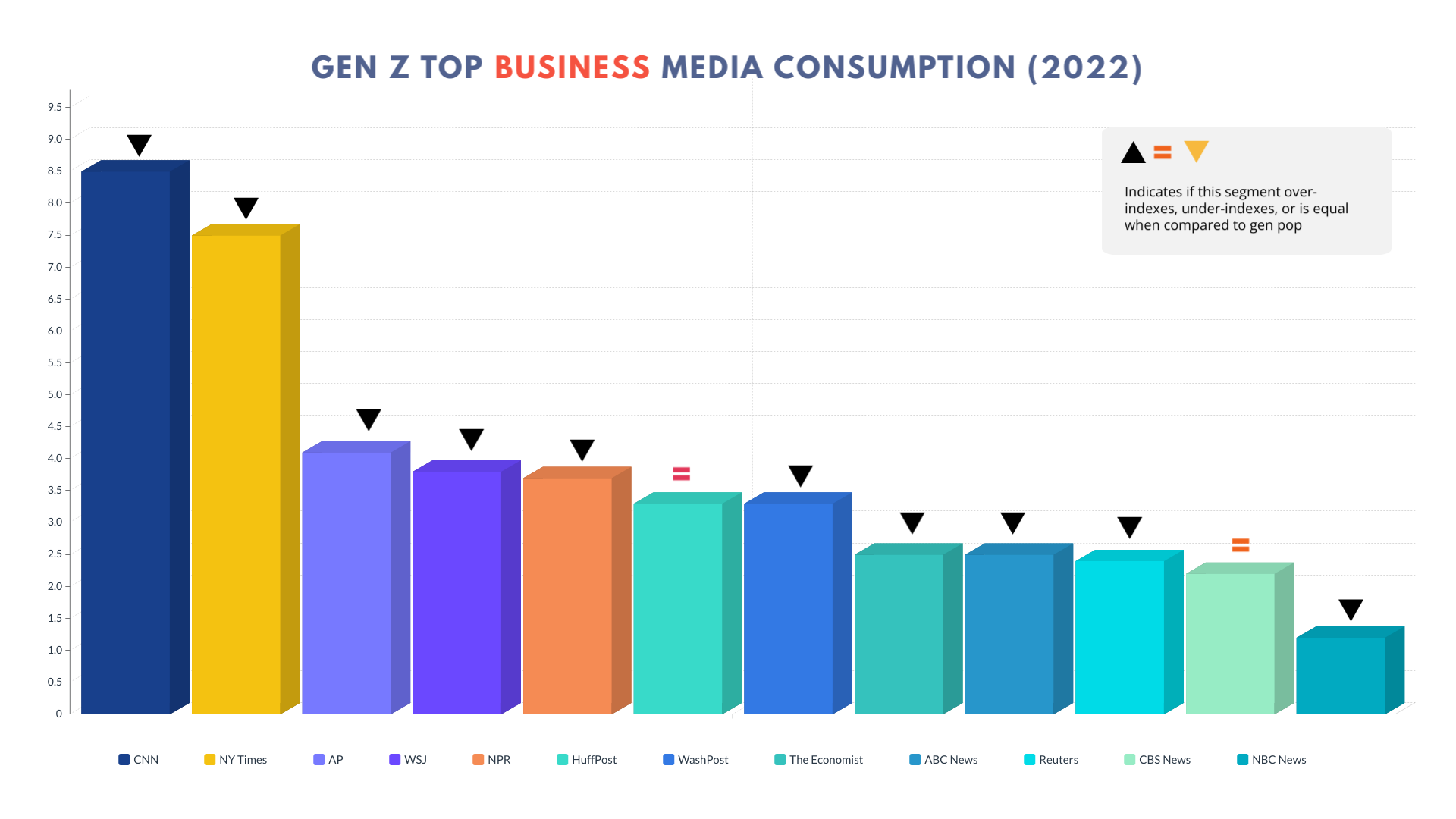This poster is a bar chart titled "Gen Z Top Business Media Consumption 2022," showcasing the preferred media outlets for Gen Z. The chart includes bars representing different media organizations, ranked from the highest to the lowest consumption, moving from left to right. The bars are displayed in varying shades of blue, purple, yellow, orange, and greenish-blue.

At the top of the chart is a tall blue bar, nearly reaching the top of the image, indicating that CNN is the most consumed media outlet among Gen Z. Following this is a slightly smaller yellow bar representing The New York Times. Next is a smaller light purple bar for the Associated Press (AP), and further bars depict other outlets such as NPR, CBS News, Reuters, and NBC News. NBC News represents the least consumed media outlet, illustrated by the smallest square in light blue at the far right. Additionally, the chart includes vertical numbers along the left side and segments showing whether the outlets over-index, under-index, or are equal compared to the general population (Gen POP). The detailed ranking and color representation provide insights into where Gen Z focuses their business media viewership.